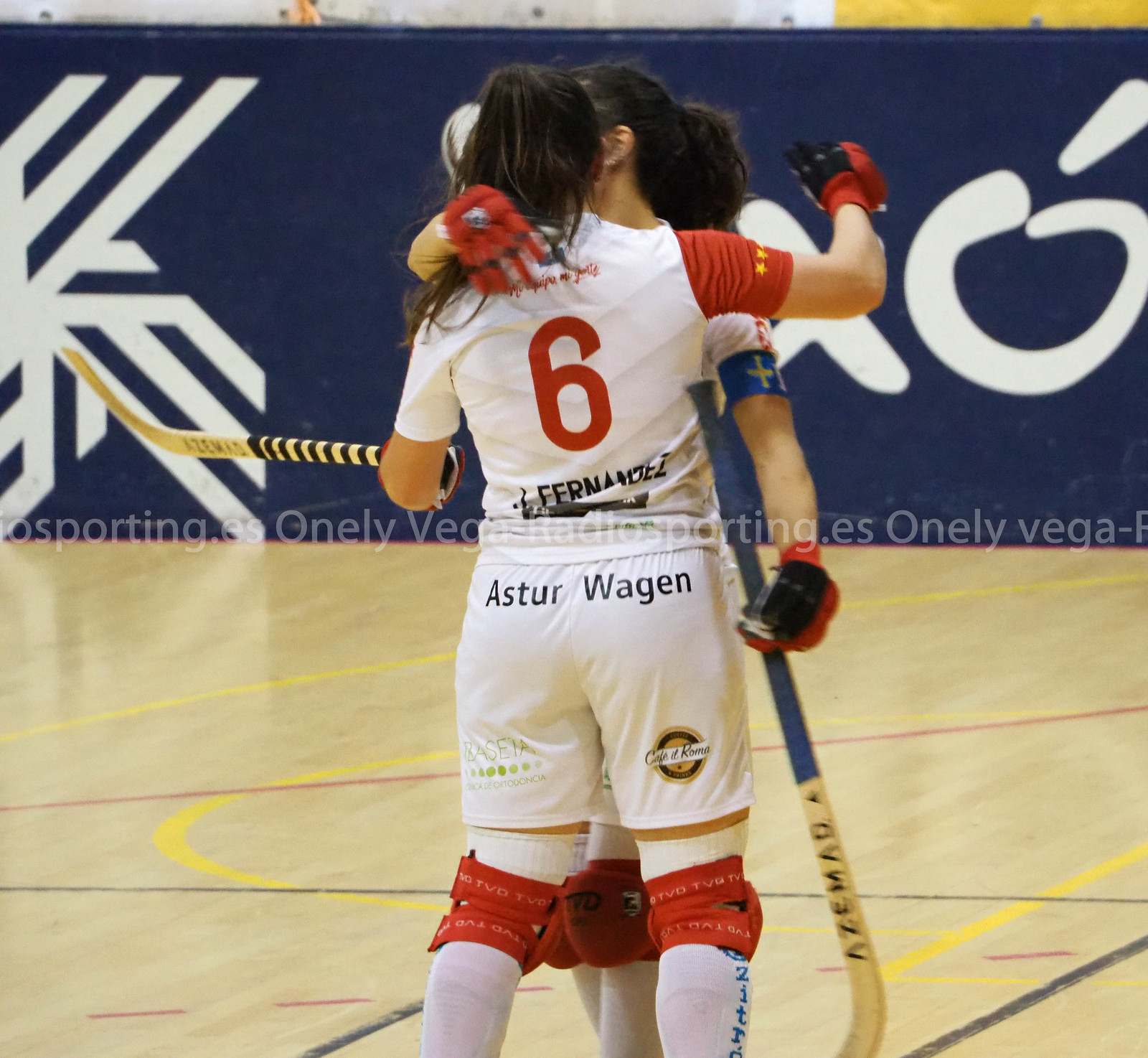In the photograph, two female field hockey players are seen hugging each other joyfully on a gymnasium court, which features a wooden floor with black, yellow, and red lines. Both athletes are dressed in white jerseys with red accents, including number six on the back of one player's uniform, which identifies her as Fernandez. The same player's shorts are marked with the name "Osterwagen" and bear a near-indistinguishable logo that seems to read "Cafe de Roma". The player being hugged, whose face is hidden, is holding a hockey stick and wearing red gloves and knee pads. Both have long dark hair tied up in ponytails. The backdrop includes a blue wall adorned with geometric white shapes, drawings, and writing. A watermark reading "Onelli Vega, Radiosporting.es" is noticeable in the middle of the image. The overall scene suggests a moment of celebration, possibly after scoring a goal or winning the game.